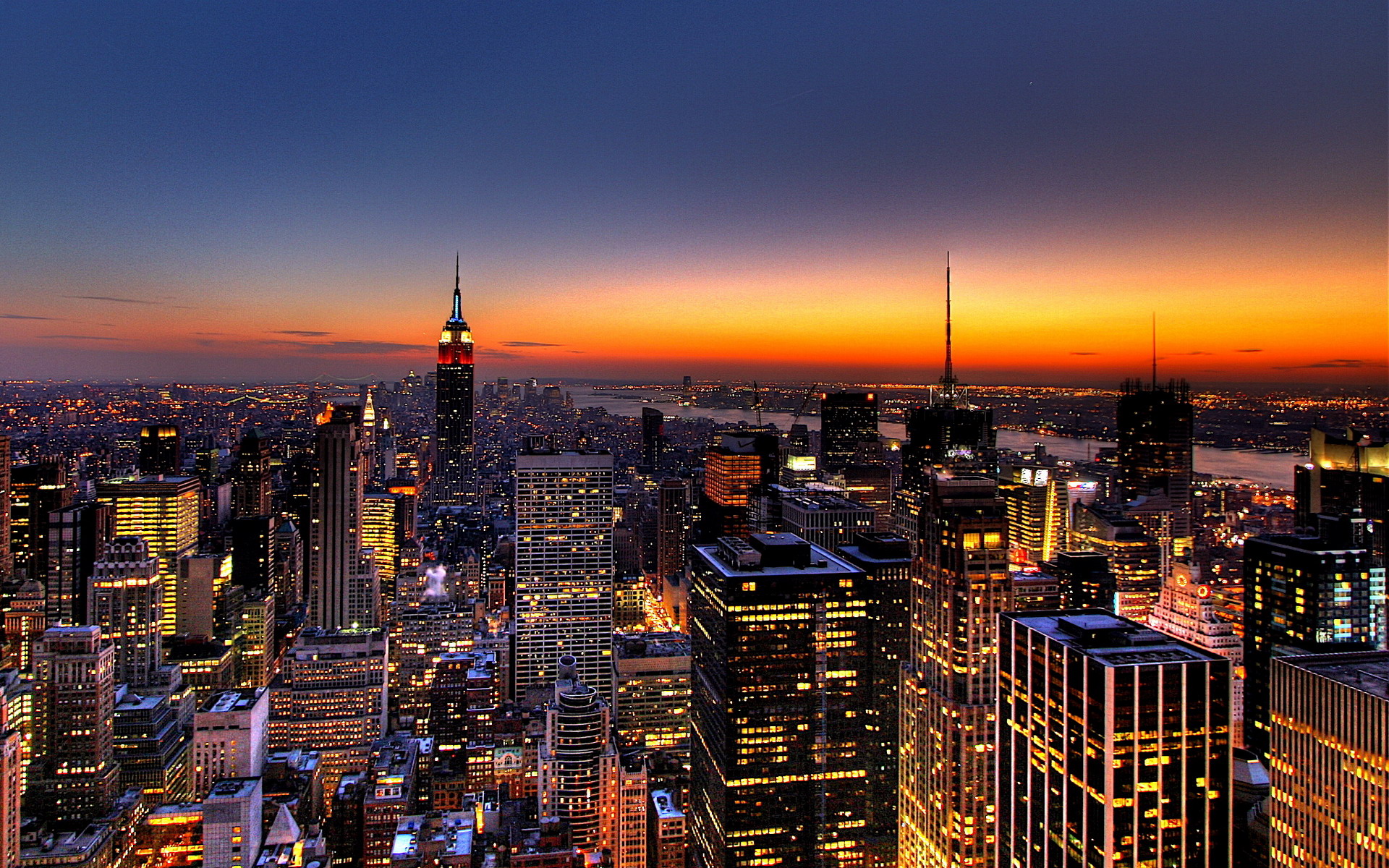This image captures a breathtaking view of the New York City skyline at sunset, seemingly taken from a high vantage point, possibly from a tall building. The sky is a stunning gradient of colors: a dark blue at the top that transitions into peach, yellow, and orange hues, with hints of blue below. The city's iconic buildings, including the Empire State Building, are prominently lit, their windows glowing with an orangish hue. The photograph offers a clear view of the sprawling cityscape, extending from the front to the distant background, where you can see shorter buildings and possibly even into the Bronx. The Hudson River, seen towards the right, reflects the sunset’s colors, creating a beautiful interplay of blue and orange. Bridges are visible in the background, connecting the city with New Jersey. The contrast of the illuminated buildings against the vibrant sunset sky makes this image an exquisite capture of New York City transitioning into night.